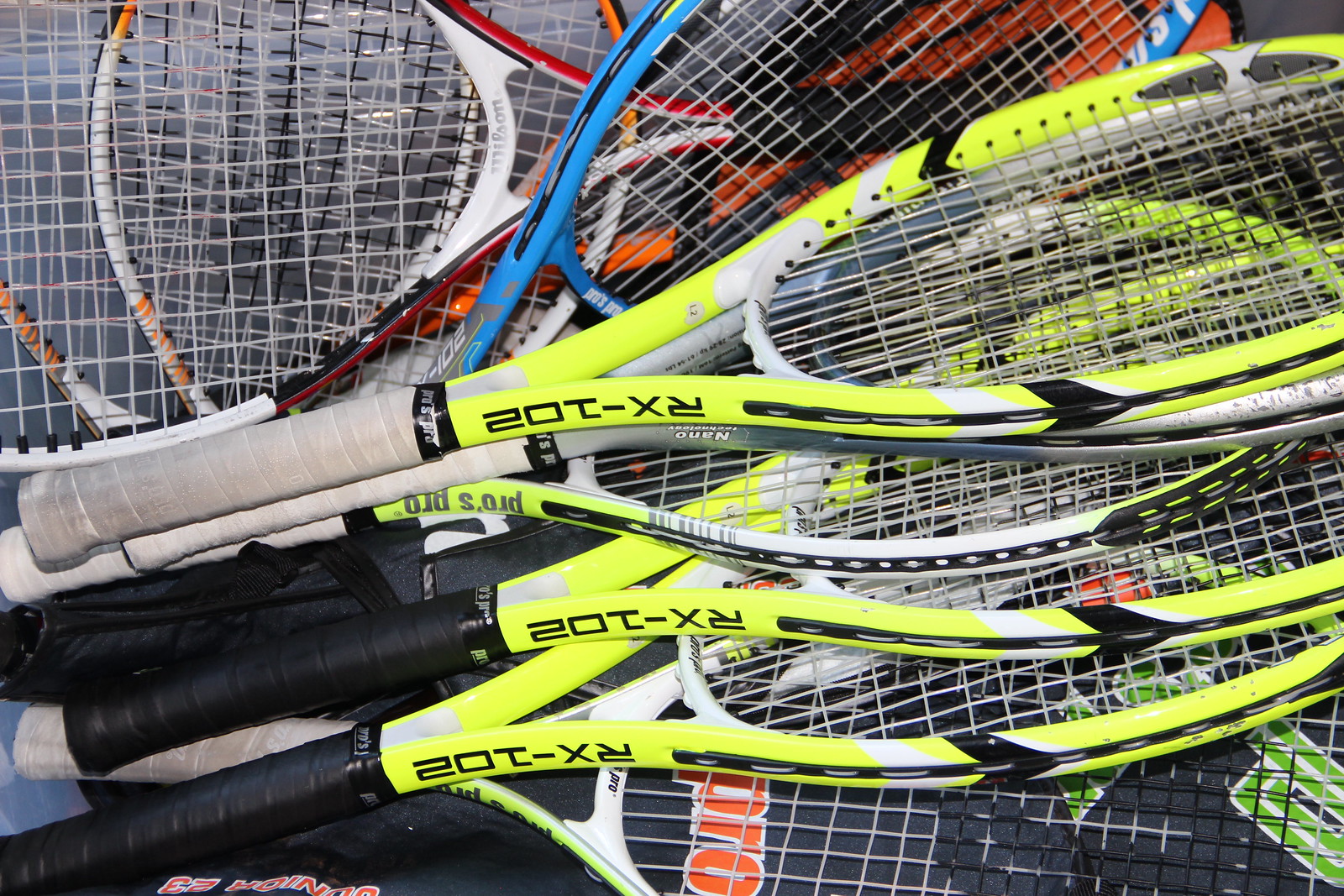This close-up photograph depicts a tightly stacked pile of tennis rackets of varying colors and conditions. Dominating the image are several neon yellow rackets with white accents, clearly marked with the model number RX-102. Their handles vary, with most being black, but there are also beige and light gray handles. Interspersed among the neon yellow rackets is a unique baby blue racket with gray accents, though its handle is obscured. Additionally, there are red and orange rackets, and one out of view, alongside some green and a few that are white. The rackets are primarily stacked with their handles pointing left and their hitting surfaces to the right, though some are oriented oppositely in the background. Most of the handles show signs of wear, with gray stitching and netting visible across the circular, almost oval-shaped frames. The background reveals a gray object, hinting at a container or cage-like setting where players might reach in to grab the rackets. Furthermore, some rackets display the brand "Pros Pro" and one simply says "Pro," indicating a mix of brands and models in this vibrant, well-used collection.